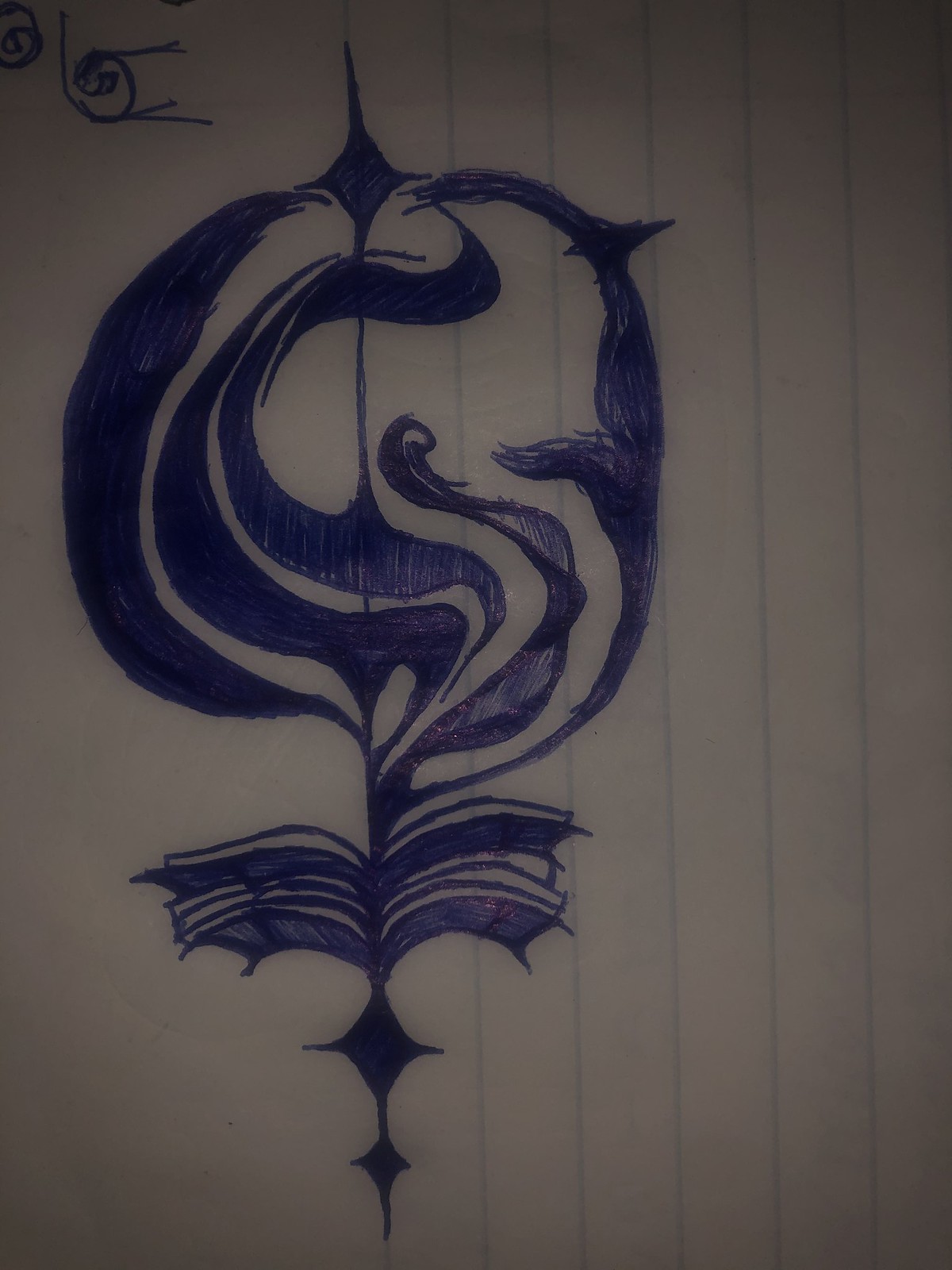This is an intricate ink doodle on off-white notebook paper with blue vertical lines. The drawing, centered along one of these lines, features an abstract composition resembling a combination of a flower and a vine. The central stem anchors the piece, with various shapes emanating from it. These include curling, ribbon-like forms creating a circular, intertwined pattern, which branch off into spiraled ribbons. Toward the bottom, diamond-shaped figures are included, adding to the detailed complexity. Throughout the piece, ribbon-like leaves flow gracefully from the central stem. Additionally, in the upper left corner, there is a small spiral with emanating lines, drawn in the same ink, enhancing the whimsical nature of the illustration.